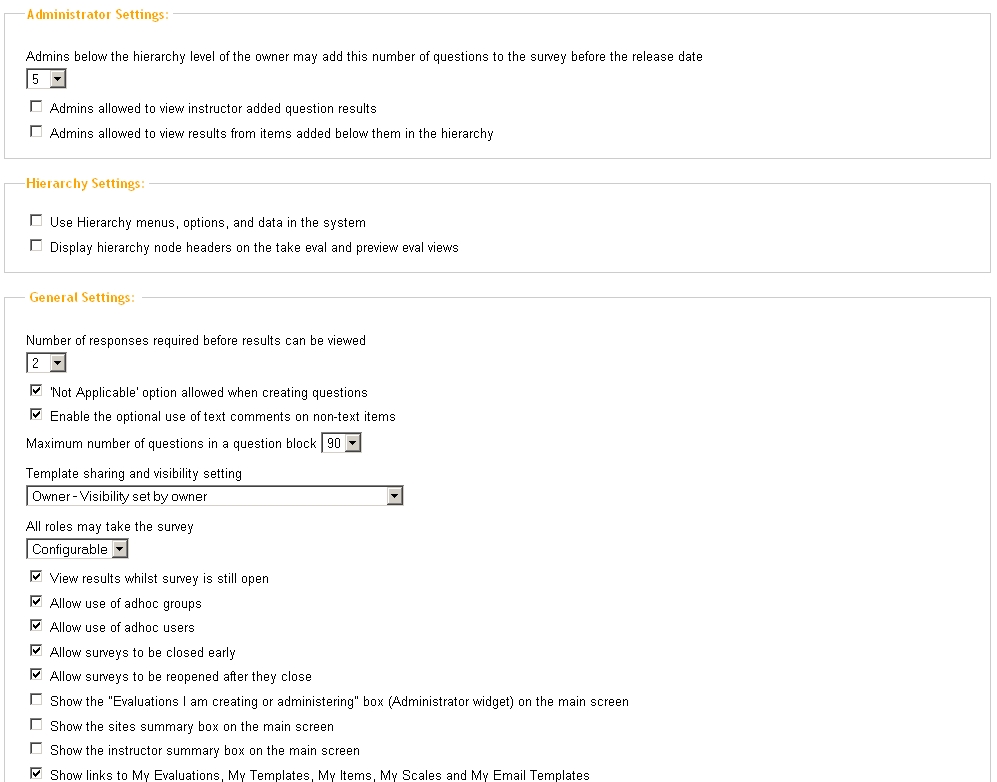**Administrator Settings Overview**

This image displays the administrative settings interface for a website or computer system, with a clean, white background. At the top, the heading "Administrator Settings" is prominently displayed. Below this, several sections and options offer an in-depth configuration of various administrative settings:

1. **Administrator Permissions:**
   - There is a section allowing administrators below the hierarchy level of the owner to add a specific number of questions to the survey before the release date, set to a value of 5.
   - Two checkboxes titled "Admins allowed to view instructor added questions" and "Admins allowed to view results from items added below to the hierarchy" are present but unchecked.

2. **Hierarchy Settings:**
   - One option titled "Use hierarchy menus, options, and data in the system" enables the use of hierarchical structures within the system.
   - Another option titled "Display Hierarchy Node Headers on the Take eval and Preview eval views" focuses on the visualization aspects during evaluation viewing and previewing phases.

3. **General Settings:**
   - The number of responses required before results can be viewed is set to 2.
   - There are two checkboxes within this section:
     - The "Not applicable option allowed when creating questions" checkbox is checked.
     - The "Enable the optional use of text commands on non-text items" checkbox is also checked.
   - The maximum number of questions in a question block is configured to be 90.

4. **Template Sharing and Visibility Settings:**
   - This section indicates that the visibility is set by the owner, with all roles potentially configurable to take the survey.

5. **Additional Viewing and Participation Options:**
   - Several settings are listed allowing for fine-tuned configuration:
     - "View Results"
     - "Allow Use of AdHoc"
     - "Allow Surveys"
     - "Show the Evals"
     - "Show the Site Summary"
     - "Show the Instructor Summary"
     - "Show Links to my Evaluation"

Each of these options is designed to manage specific administrative functionalities and permissions, ensuring a customizable and controlled environment for managing surveys, evaluations, and hierarchy data display.